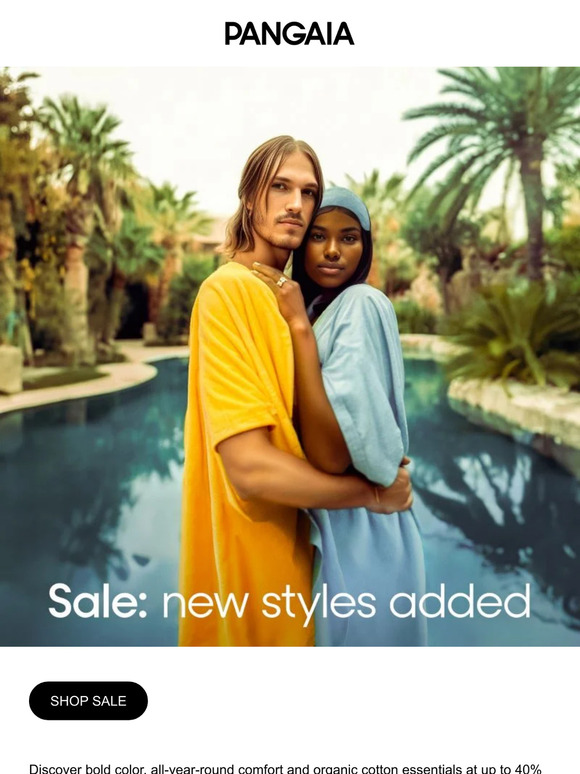Here is a cleaned-up and detailed caption for the described image:

---

"This advertisement, with a sleek white background, prominently displays the brand name 'Pen Letters' at the top. Featured in the center is a large, vibrant photograph capturing a man and woman in a warm, affectionate hug beside a sparkling pool framed by lush palm trees. Both individuals are dressed in cozy, white terrycloth gowns. The man, who has long blonde hair, and the woman, whose long black hair is neatly kept back with a matching terrycloth headband, gaze directly into the camera, exuding a sense of relaxation and intimacy.

Below this heartwarming image, bold white lettering announces a 'Sale,' with 'New Styles Added' situated just to the right. Positioned to the left beneath the photo, a striking black button labeled 'Shop Sale' in white text invites viewers to explore the offerings. At the very bottom of the ad, small black text encourages shoppers to 'discover bold color, all-year-round comfort, and organic cotton essentials at up to 40% off,' although the message is cut off at this point."

---